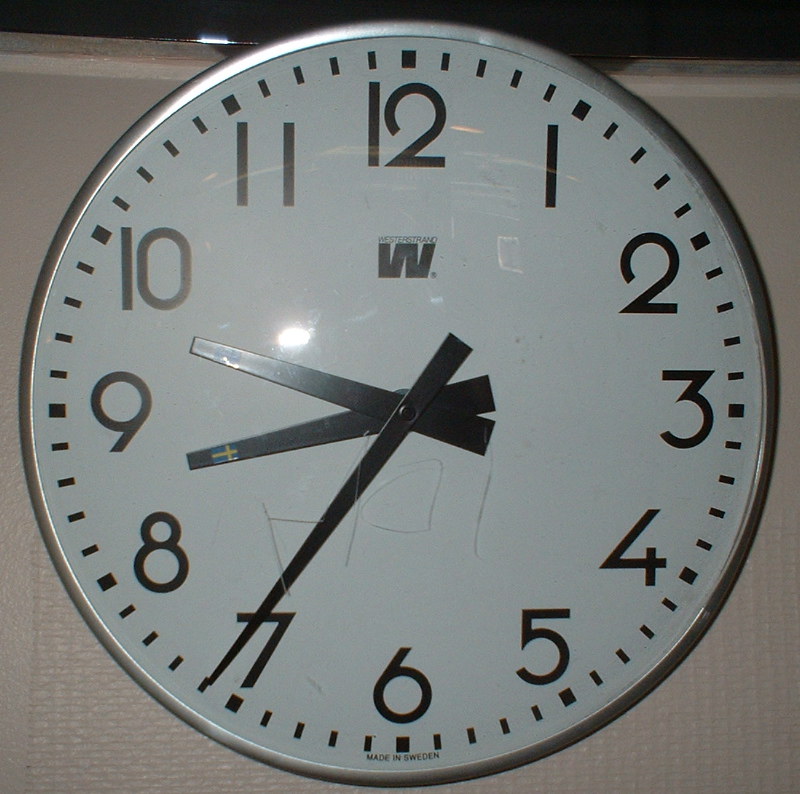A close-up photograph of a classic analog clock with a sleek silver rim and a pristine white face. The clock features black Arabic numerals, arranged traditionally from 1 to 12, and fine black minute ticks between the numbers. Three hands are visible: the hour hand is just past the 8, the minute hand is slightly past the 9, indicating approximately 8:47. The slender, longer second hand, also in black, is positioned just past the 7. The clock's surface shows a few visible scratches. The background is a simple gray, suggesting the clock is mounted against a small, unobtrusive wall.